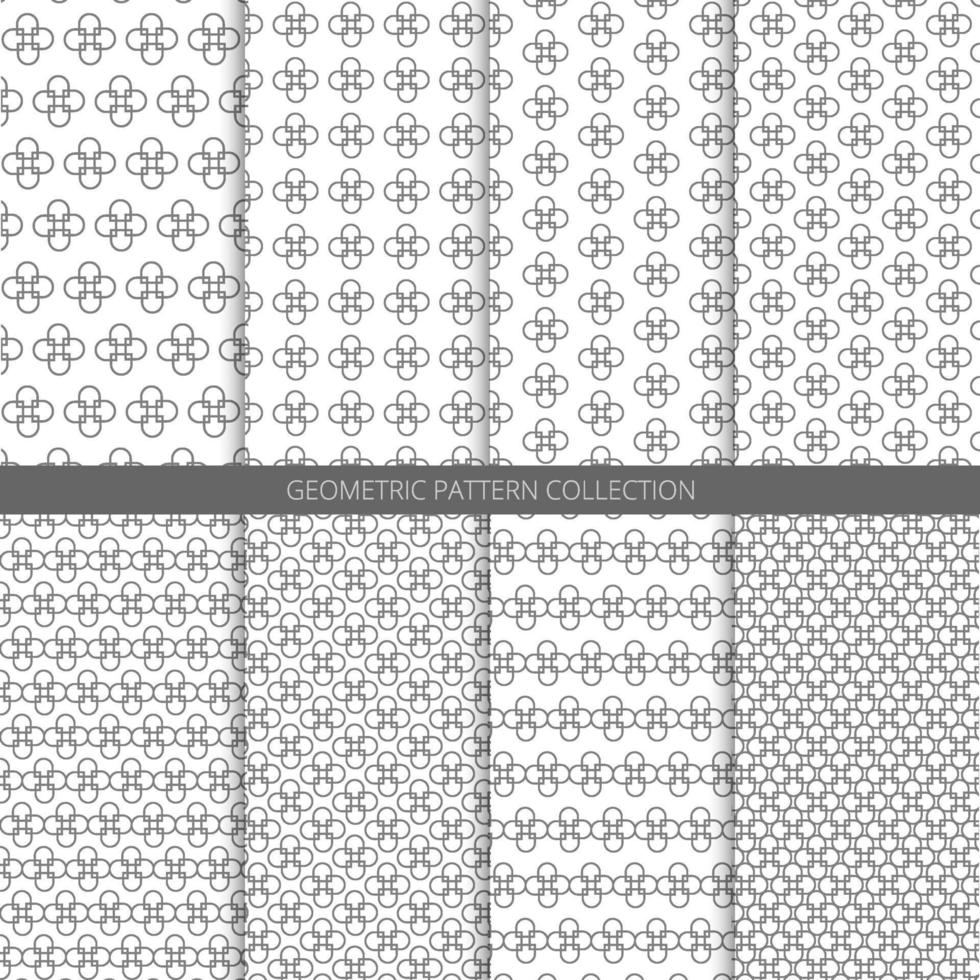The image titled "Geometric Pattern Collection" features eight distinct geometric patterns displayed in vertical rectangles with a white background and gray designs. A central gray banner runs horizontally across the middle of the image, bearing the title in white text. Each pattern consists of repeating shapes that resemble four interconnected half-circles or semi-circles, oriented to form clover-like or floral designs. These designs vary in density and arrangement:

1. **Top Left**: The shapes are sparsely spaced, arranged in alternating rows.
2. **Top Center-Left**: The shapes are regularly spaced without row shifts.
3. **Top Center-Right**: Similar shapes are shifted every other vertical line, appearing larger.
4. **Top Right**: Shapes are also shifted vertically and enlarged.
5. **Bottom Left**: Shapes touch tangentially and alternate every other row.
6. **Bottom Center-Left**: Arranged in a 45-degree diagonal grid.
7. **Bottom Center-Right**: Tangentially touching and alternated horizontally, but with wider spacing.
8. **Bottom Right**: Densely packed, creating a seamless grid-like appearance with no white space between shapes.

Overall, the patterns range from loose and spacious to tightly compacted, showcasing different geometric arrangements of a consistent design motif.